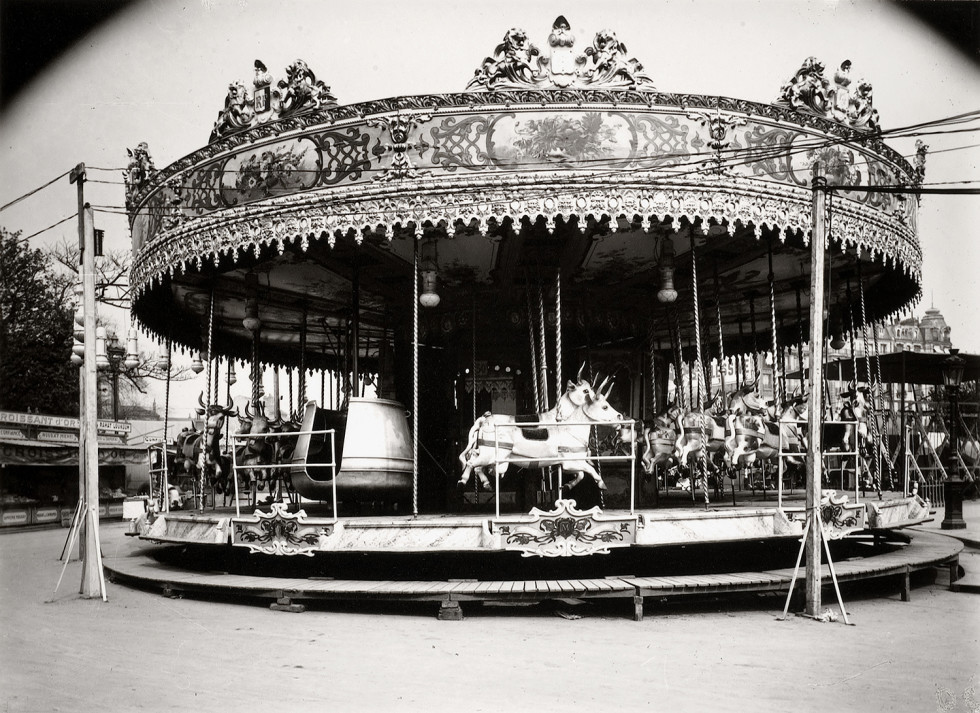The image is a black and white photograph, possibly from an older era, depicting an intricate carousel, likely set in a carnival or circus. Central to the image are two white cows mounted on poles that spiral downwards, adorned with black saddles and horns pointing upwards, their front legs reaching forward and back legs extended behind, giving the impression of motion. Above the cows, the carousel features an ornate circular canopy with sharp, intricately designed points hanging down. The top section of the carousel displays images of trees, and at the very peak, there's a gnome-like figure with a dark hat surrounded by floral designs set against a white half-circle that resembles a rising moon.

In addition to the carousel, the scene includes other fair attractions visible in the background, including a building with a turret-like top to the center right and what appears to be sideshow games on the left. The carousel is enclosed by a wooden walkway composed of planks that fully circles the ride, and two poles with wires run across the top center of the image. The detailed and ornamental decorations on both the top and bottom of the carousel, along with the utility lines and additional rides and amusements in the background, further contribute to the vintage and festive atmosphere captured in this photograph.